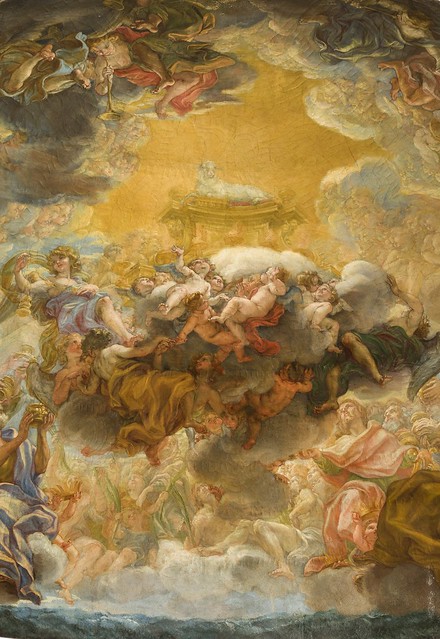The painting is an elaborate depiction teeming with figures arranged around a central focal point. At the top corners, stormy gray clouds swirl with robed individuals flying within them, including one playing a horn. These clouds part to reveal a radiant golden sky, where a majestic gold pedestal with a red velvet cushion sits, crowned by a white-woolen sheep gazing solemnly down.

Beneath this celestial platform, a ring of children and robed figures look up towards the sheep in awe. Further below, more adults in robes and armor also direct their gazes upward, adding to the painting's grandeur and depth. The scene blends elements of heaven and earth, possibly illustrating the transition of man to a divine realm. Various shades of white, brown, red, yellow, pink, and orange interweave to create a rich, complex tapestry of colors and emotions, with figures of all ages and conditions – some cloaked, some bare, and all in a state of reverent observation.